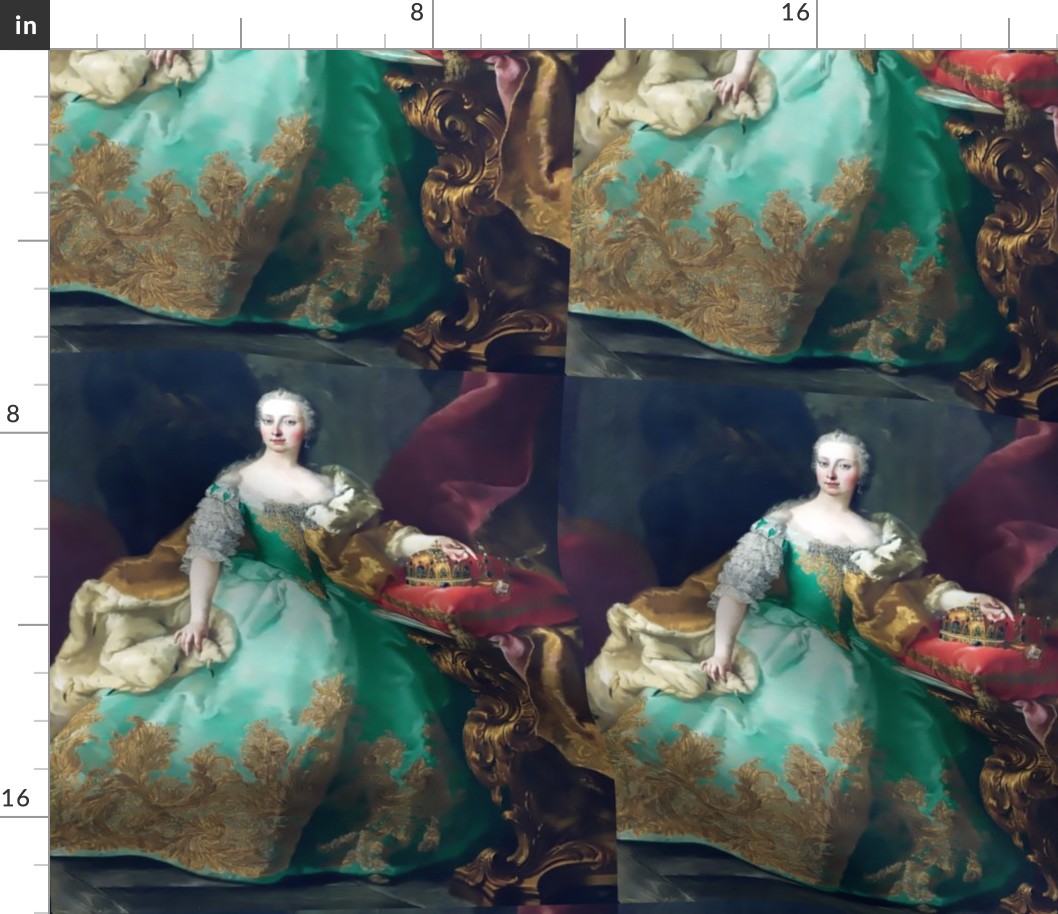This photograph appears to depict a Victorian-era painting, presented in a unique four-panel format where each panel showcases different portions of the same image. The central figure is a distinguished woman clad in a voluminous green Victorian dress adorned with gold leaf-like patterns at the bottom and up the corset. Her attire includes frilly arm sleeves that add to the elaborate ensemble. Her cheeks are subtly reddened, hinting at makeup, while her hair is neatly tied back, revealing her face. 

The woman is seated, possibly on a bed or large chair, with a lush blanket positioned over her right side, held by her right hand. Her left hand rests elegantly on a red cushion placed atop a carved wooden podium, and on this cushion sits a crown, suggesting her royal status, potentially representing a figure like Catherine the Great. 

In the individual panels, subtle variations are visible: the lower left panel aligns closely with the central image but with a differently positioned armrest, which is gold with a lion motif; the upper left panel shifts focus to show more of the armrest's gold base; the upper right shows details of her dress and part of the armrest. An additional measurement marker in white text can be seen along the edge of the photograph, denoting 8 and 16 inches both horizontally and vertically. 

Overall, the composite image conveys a regal aura, capturing the richness and intricacy of Victorian royal fashion.